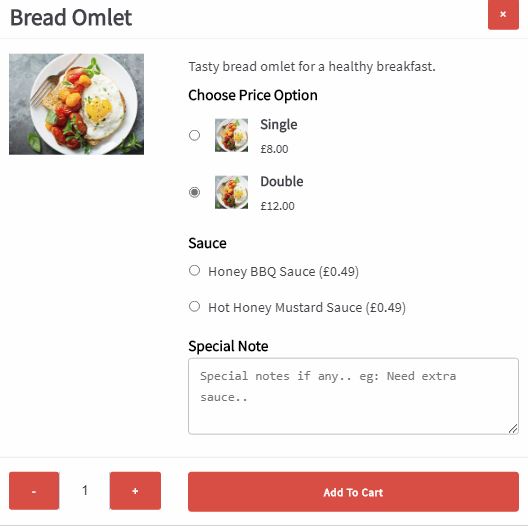The image appears to be a screenshot or photograph taken from within a food delivery or ordering app. At the very top, on a white background, there's a search bar located on the upper left corner with the text "Bread Omelette" in black lettering. On the far right side of the search bar is a red box containing a white "X".

Directly below the search bar, there is a square image displaying a meal: a white plate with eggs positioned on the right side and what appears to be potatoes on the left side. A silver fork is placed at approximately the 11 o'clock position on the plate.

Underneath the image, in bold text, it reads "Tasty Bread Omelette for a healthy breakfast." Following this description, "Choose price option" is also bolded in black.

Two identical images, showing the same meal described earlier, are displayed beneath this text. Each image has a corresponding radio button to the left. The first option, labeled as "Single," is priced at 8 pounds and is not selected. The second option, labeled as "Double," is priced at 12 pounds and is selected.

Below these options, there are sauce choices listed: "Honey Barbecue Sauce for 49 cents" and "Hot Honey Mustard Sauce for 49 cents." Each sauce option also has a radio button beside it, but neither are selected.

At the bottom of the image, there is a text field titled "Special Note" where additional comments or instructions can be entered. 

Spanning across the bottom of the screen, there is a quantity selector composed of three elements: a square red button with a white minus sign on the left, a number "1" on a white background in the center, and a square red button with a white plus sign on the right. To the immediate right, there is a long rectangular red button with the text "Add to Cart" in white.